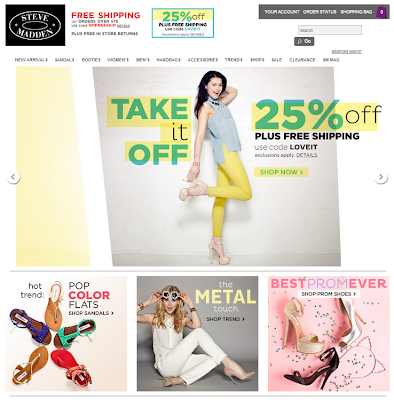The image displays a shopping web page featuring a vibrant collection of fashion items. The main section highlights a woman showcasing a pair of nude-colored high-heeled pumps. She is dressed in yellow pants and a light pastel blue sleeveless blouse, and has dark hair. The woman is posed with her right leg bent at the knee, gracefully touching the heel of her shoe. Prominent green text on a yellow background flanks her image, announcing a "Take 25% Off" sale with the prompts "Take it off" and "Shop now."

Below this central image, there are additional images of footwear. On the left side, an array of shoes is displayed in green, red, brown, and blue hues. Adjacent to these shoes, the text reads "Pop Color Flats." On the right side of the main image, more shoes are showcased, accompanied by the caption "Shop Sandals."